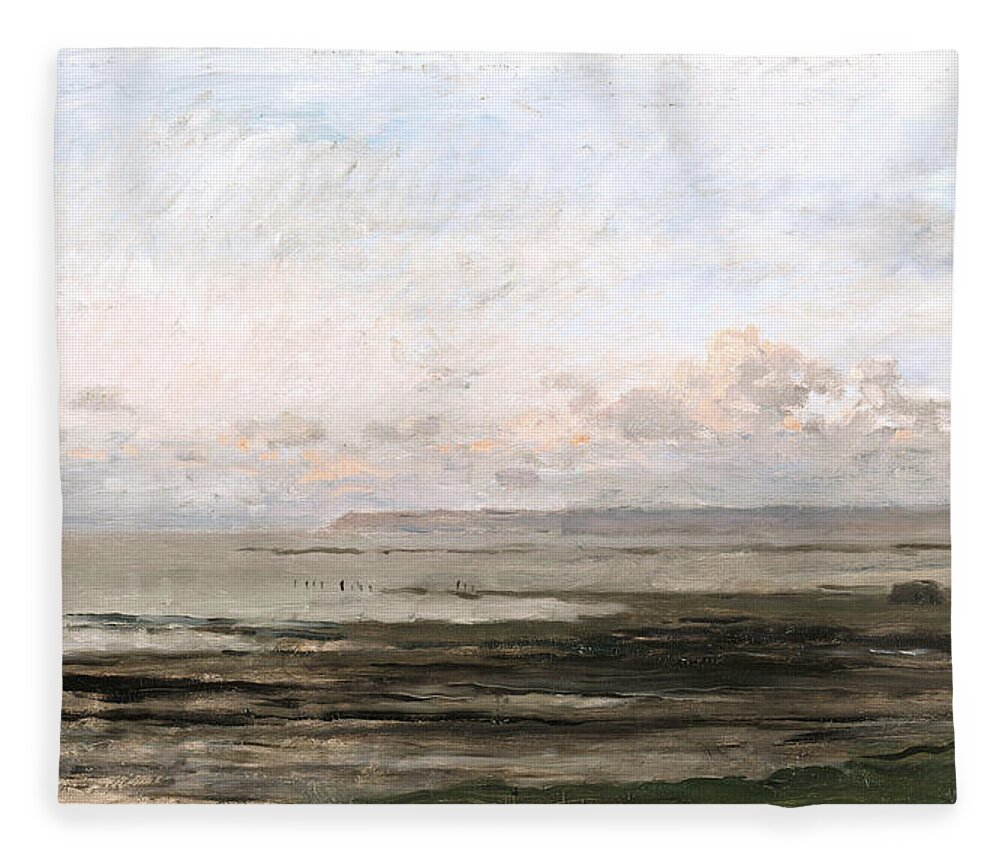In this painting, set on a canvas stretched over a frame, the scene depicts expansive, desolate plains rendered primarily in desaturated tones of dull browns, greys, and hints of blues. The landscape, possibly a dried lake bed or salt flat, is vast and flat, with no grass or vegetation. The horizon line sits about a third of the way up the image, marking the transition to a sky filled with a mix of thicker clouds and sparse blue patches. In the far distance, one can discern a small plateau and a faint silhouette of a mountain. Across the plains, the faint outlines of stick-figure people walk, emphasizing the emptiness and isolation of the landscape. Despite the simplicity of the palette and composition, the artist skillfully conveys a sense of melancholy and abandonment through the sparse use of warm blues and the overall desaturated tones.